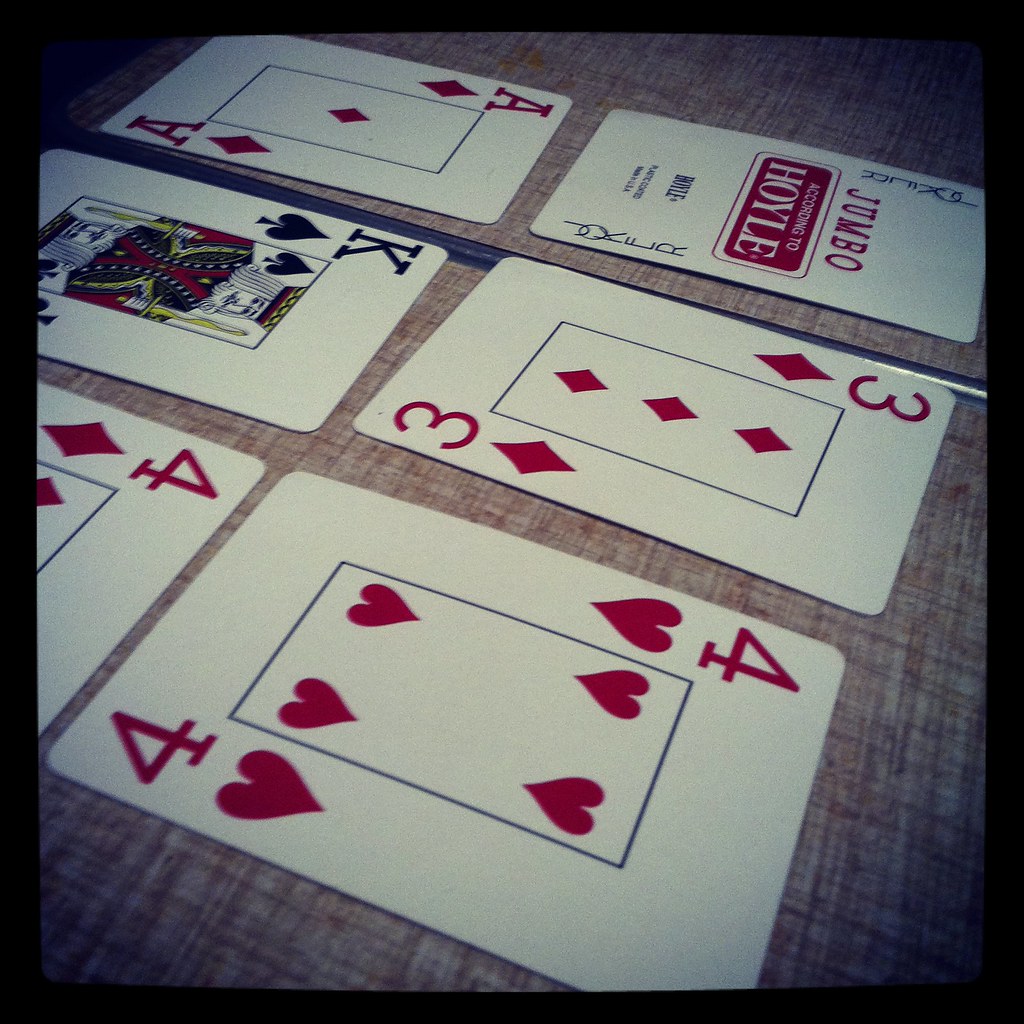A square photograph, encased in a black frame, captures a close-up view of six playing cards arranged on a cross-hatched surface. The lighting is dim, focusing solely on the cards, casting the surroundings into shadow. The playing cards are displayed face-up in two rows of three, angled at approximately 45 degrees from the bottom left to the top right. 

In the bottom row, viewers see a four of hearts, centered by a three of diamonds, with a joker card completing the sequence on the right. The top row consists of a four of diamonds on the left, a king of spades in the middle, and an ace of diamonds on the right. Although not perfectly aligned, the cards are placed close together, creating a unified yet slightly offset visual effect. The image is artistically vignetted, with each corner fading to black, emphasizing the illuminated playing cards at the center and enhancing the dramatic focus on the subject.